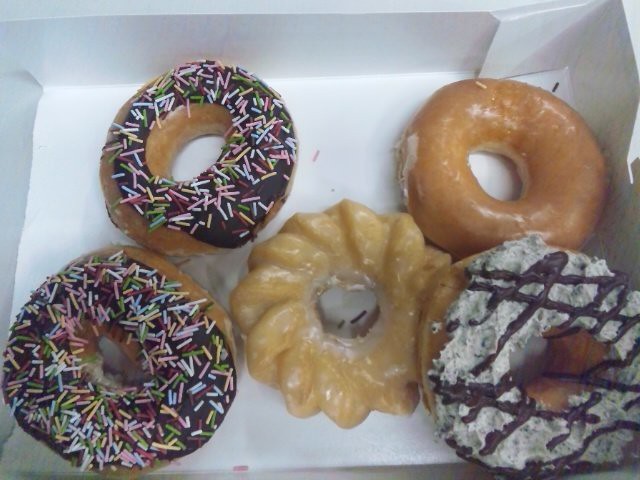This image is a close-up, top-down view of a white cardboard box containing five doughnuts, arranged in an X pattern. The box, typically used for doughnuts, has one doughnut in the center and four situated in each corner. 

On the left-hand side, there are two identical raised yeast doughnuts with a ring of chocolate frosting and a generous helping of colorful rainbow sprinkles (pink, red, green, yellow, and white) on top. 

The doughnut in the center is an old-fashioned style, featuring raised ridges and covered with a smooth glaze. 

In the top right corner, there's a standard raised glazed doughnut with a conventional smooth surface.

The bottom right corner holds a unique doughnut that appears to be topped with white frosting crisscrossed with chocolate, likely hinting at a cookies-and-cream flavor due to its white and black speckling.